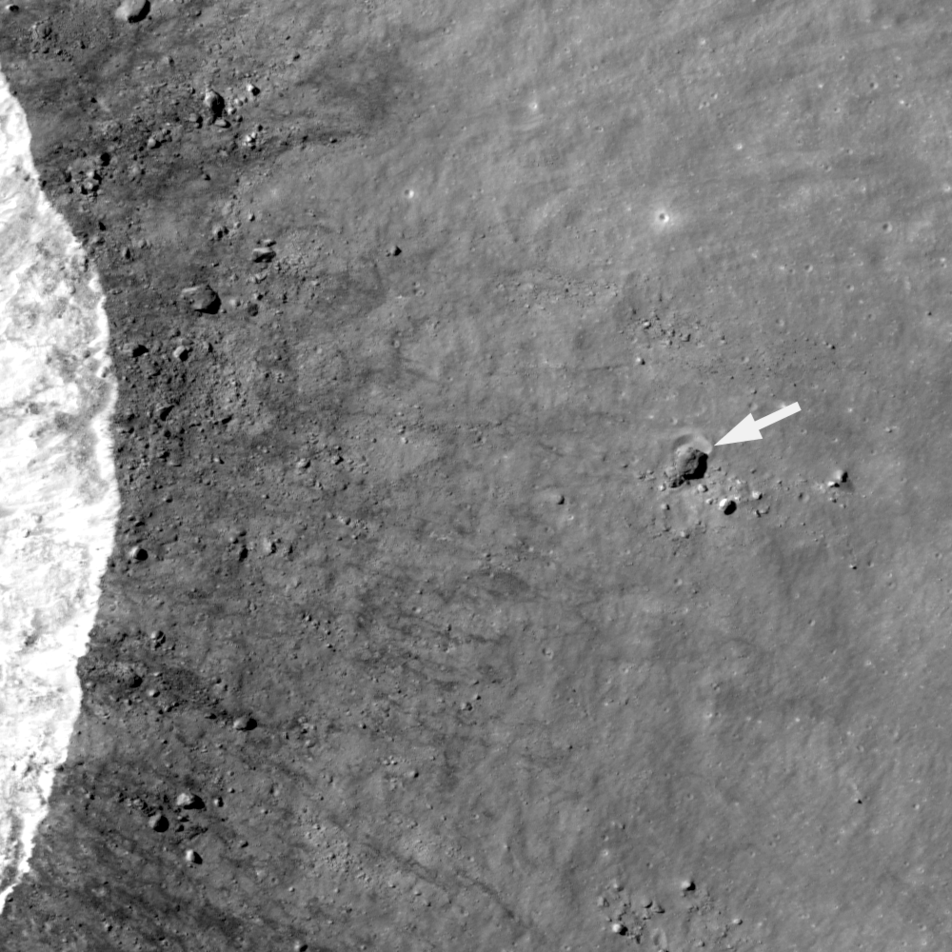This black-and-white image captures a close-up of a rocky, moon-like surface. Predominantly gray, the right side of the picture features scattered tiny rocks and specks that resemble gravel or dirt. A significant detail is a rock in the middle-right section of the image, marked by a white arrow pointing towards it. The left side of the picture contains a semi-circular white area, contrasting sharply with the rest of the terrain, adding a point of interest to the otherwise monochromatic scene. The surface also displays numerous small holes and uneven textures, highlighting its rugged nature. This detailed view, filled with dirt, rocks, and surface irregularities, could represent either a part of the Earth's landscape or a simulation of the lunar surface.